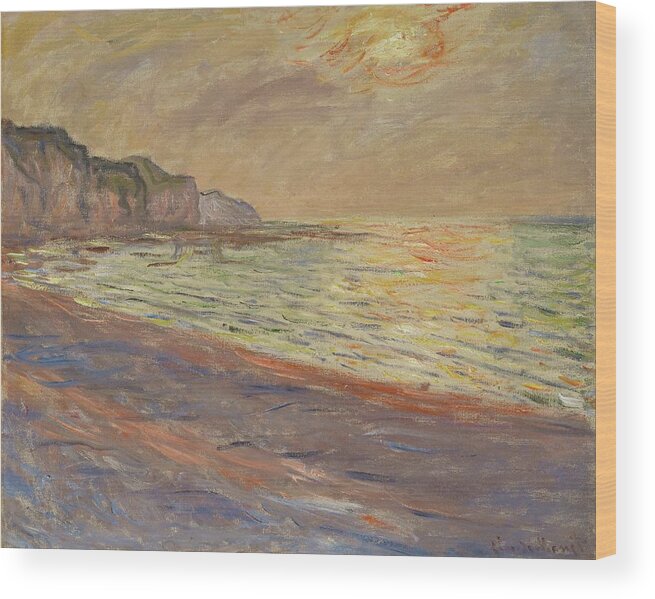The painting on canvas, seemingly created in an impressionist style, depicts a coastal landscape. The sand of the beach features a blend of brown, gray, and blue strokes, giving it a textured appearance. The water is rendered with strokes of green and blue, accented by the golden and orange reflections of the sun, which is positioned high on the canvas, casting its light. The sky above boasts a swirl of gray, peach, and mustard hues, suggesting a sunset or an overcast day. On the left side of the horizon, there are cliffs or rocky outcroppings, contrasting with the clear expanse of open sea. The canvas itself has a blonde wood finish along the edges and is displayed on a white wall, adding a touch of refined simplicity to the overall presentation. The distant shoreline curves gently, dominated by more subdued tones of rusty browns and blues, emphasizing the rugged nature of the beach rather than a light, sandy appearance.